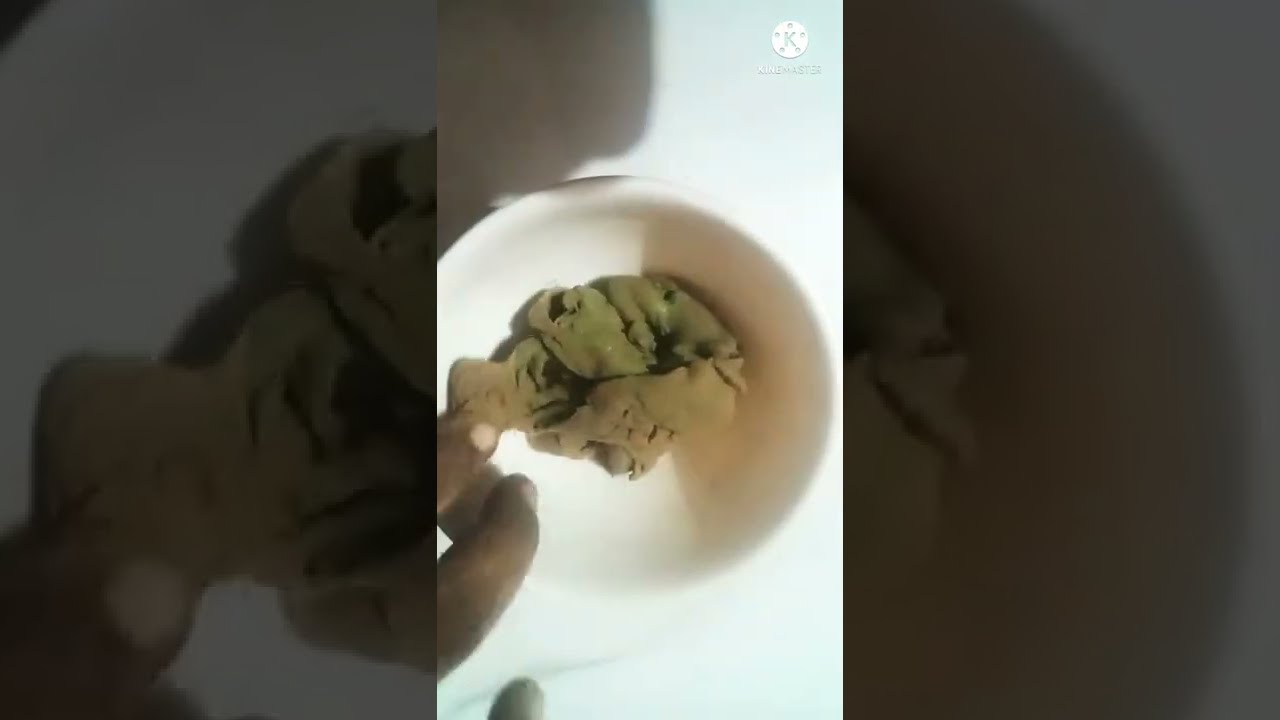The image depicts a small white bowl containing a mysterious greenish-brown mixture, possibly resembling algae or clay, or even a scoop of dark ice cream. Brown-skinned fingers are seen poking at the content in the bowl. The photograph, framed with neutrals—black, white, brown, tan, off-white, and olive green—showcases a logo at the top featuring a circle with a "K" in it, alongside some indistinguishable letters below. The picture appears to be divided into thirds; the left and right thirds are dark and blurry, giving the effect of looking through a filter, while the middle third is brighter, providing a clearer view of the bowl and its contents. In the background, there is an enlarged, darker version of the main image, contributing to the overall complex and somewhat abstract composition. The setting is against a white background, emphasizing the focus on the bowl and the hand interacting with it.